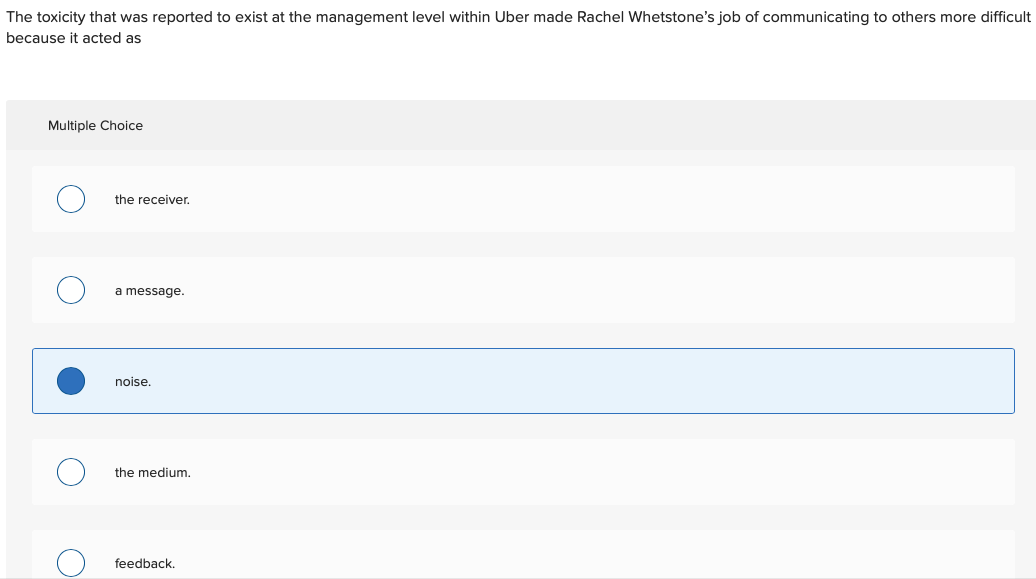The image features a white background illustrating the challenging communication dynamics at Uber, specifically at the management level. It highlights the obstacles faced by Rachel Whetstone, whose job of conveying messages was impeded by reported toxicity within the company. This complexity is visually represented through a diagram. 

At the center of the image is a gray box displaying multiple-choice elements. Each element represents a different component of the communication process. Alongside the gray box, there are five accompanying terms: "Message," "Noise," "Medium," "Feedback," and "Receiver." Each term is marked with an unshaded circle, except for "Noise," which is distinguished with a shaded blue circle, emphasizing the disruptive role of noise in effective communication. 

This conceptual visualization effectively captures the intricate barriers within Uber that interfered with the seamless transmission of information under Rachel Whetstone's oversight.